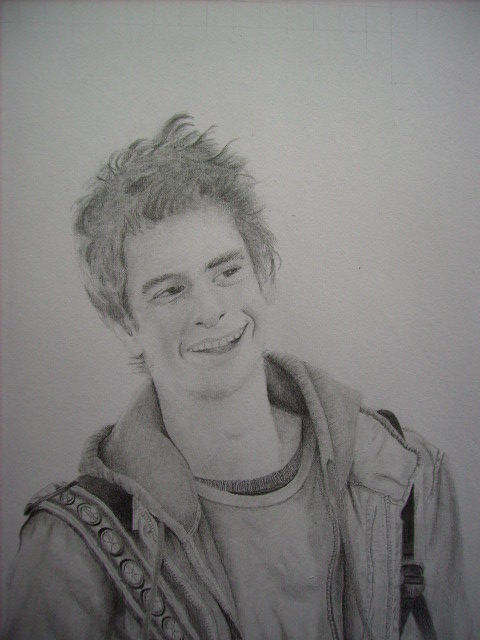This black-and-white image, resembling a sketch or a pencil drawing, portrays a young white male from the chest up, positioned vertically in a rectangular frame. He sports a wide, toothy smile, possibly laughing, with visible tongue and deep creases at the corners of his mouth. His head leans slightly to the left, and he gazes off to the right. The young man has medium-length, somewhat messy hair, styled with a lot of hairspray or gel, spiking upwards and outwards, partially covering his ears.

He is dressed in a layered fashion, wearing a jacket with a hood, over two shirts – the top shirt being slightly lighter than the bottom. His attire is further detailed with a strap hanging from each shoulder; the one on the left appears to be a plain black strap, whereas the strap on the right has a wider, decorative, geometric pattern. The background of the photo is a light shade of gray, adding to the overall impression of a meticulously detailed pencil sketch despite the lack of color.